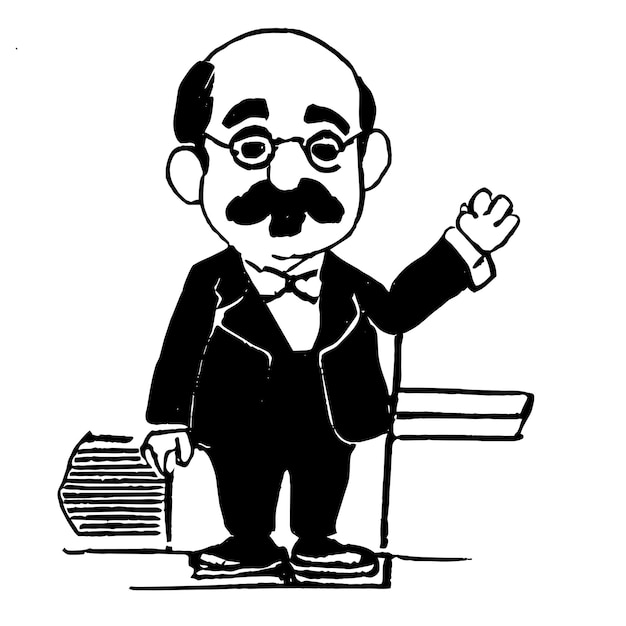The image is a detailed black and white drawing of a man who appears to be in his 60s. He has a partly bald head with hair on the sides and thick black eyebrows. He sports a large, thick mustache and wears black spectacles. The man is dressed in a black suit with black pants, black shoes, and a white tie. His left hand is raised as if waving, while his right hand rests by his side. His expression is calm and somewhat expressionless. The background of the image is white, featuring a box-like structure on the left and some black lines on the right, possibly depicting a podium with a side tray and grate, suggesting he might be an instructor or director.